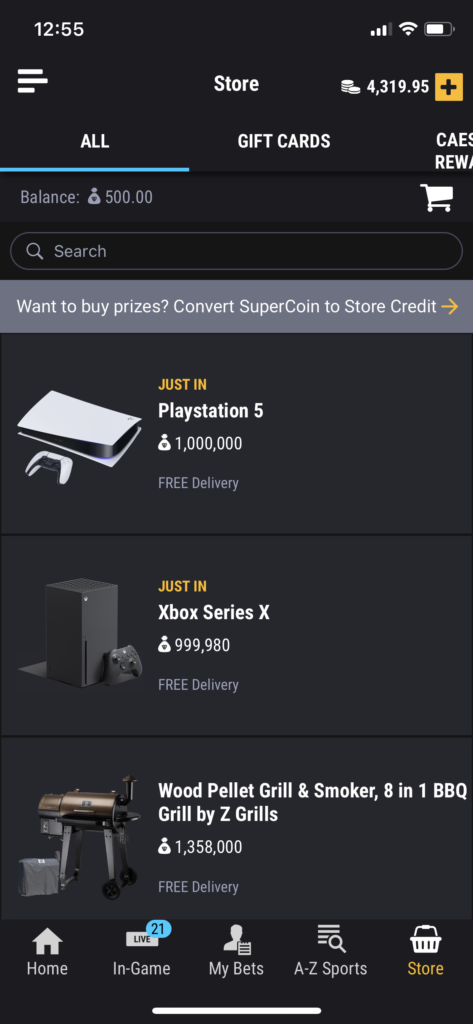The image displays a mobile website on an Android phone, which appears to be in dark mode. The background is entirely black. At the very top of the screen is the "Store" tab. Below this, there are several categories including "All," "Gift Cards," and "Reviews." The current view is the shopping cart.

In the shopping cart, a message appears stating, "One of my prizes converts supercoin to store credit." 

Below this message, there are several items listed in the cart:
1. **PlayStation 5**: The listing includes an image of the PS5 and text reading "Just in: PlayStation 5 for 1,000 - Free delivery."
2. **Xbox Series X**: This item also has an accompanying image and the text "Just in: Xbox Series X 999 and 980 - Free delivery."
3. **8-in-1 Wood Pellet Grill and Smoker by Seagrills**: A picture of the grill is shown, along with its description and the price "1,358,000 - Free delivery."

At the bottom of the screen, there are several navigation icons:
1. **Home** icon
2. **In-Game/Live** icon with 21 notifications
3. **My Bets** icon marked by a person's head
4. **A to Z Sports** icon with a magnifying glass
5. **Store** icon marked by a shopping basket

The interface appears succinct, containing various shopping and navigation elements geared towards a comprehensive browsing and user experience.